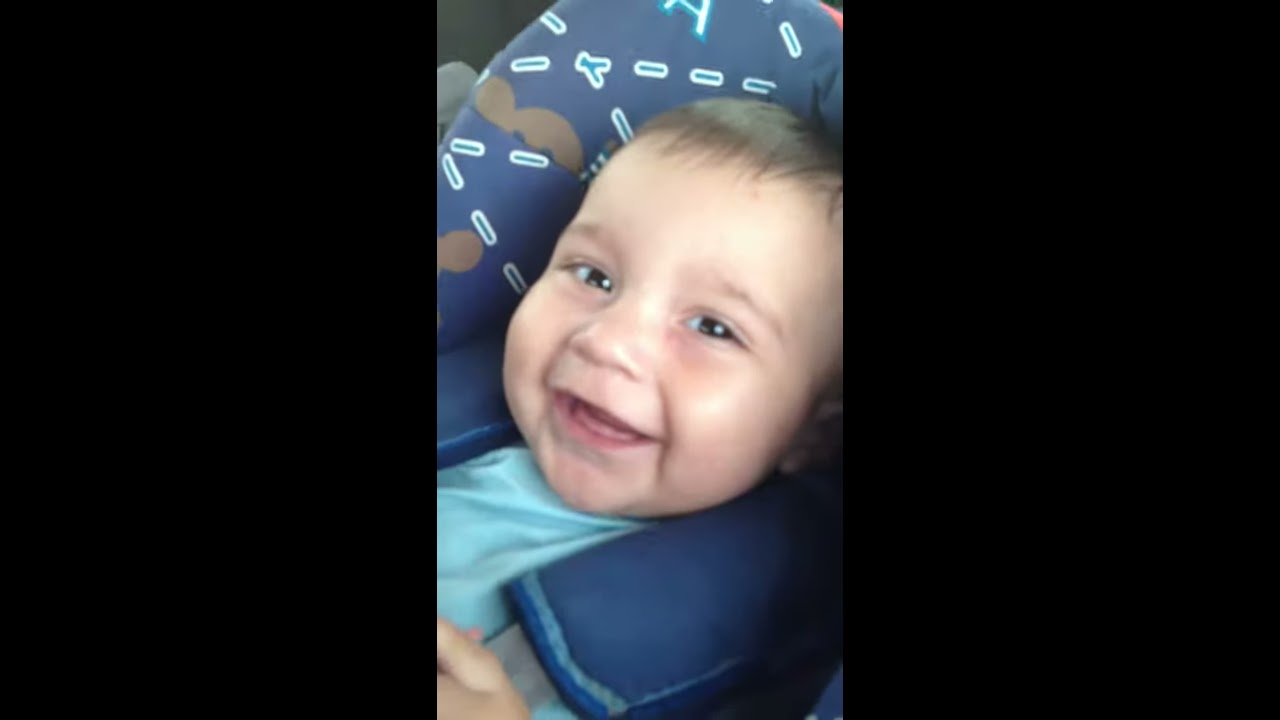This digital photograph features a close-up of a smiling baby, likely a boy, who appears to be between a few months to a year old. The baby has dark hair and light brown eyes, with chubby cheeks that accentuate his cheerful expression. He is seated in a car seat, which has a dark blue back panel with lighter blue markings resembling a 'Y' and some dashes. The straps of the car seat, which are also dark blue, secure him in place. He is wearing a light blue shirt, and a bit of his hand is visible in the frame. The car seat's padding surrounds his head, and there is no text, only decorative designs on the seat. The baby is the sole focus of the image, with no other people or objects visible in the background, and the setting appears to be indoors.